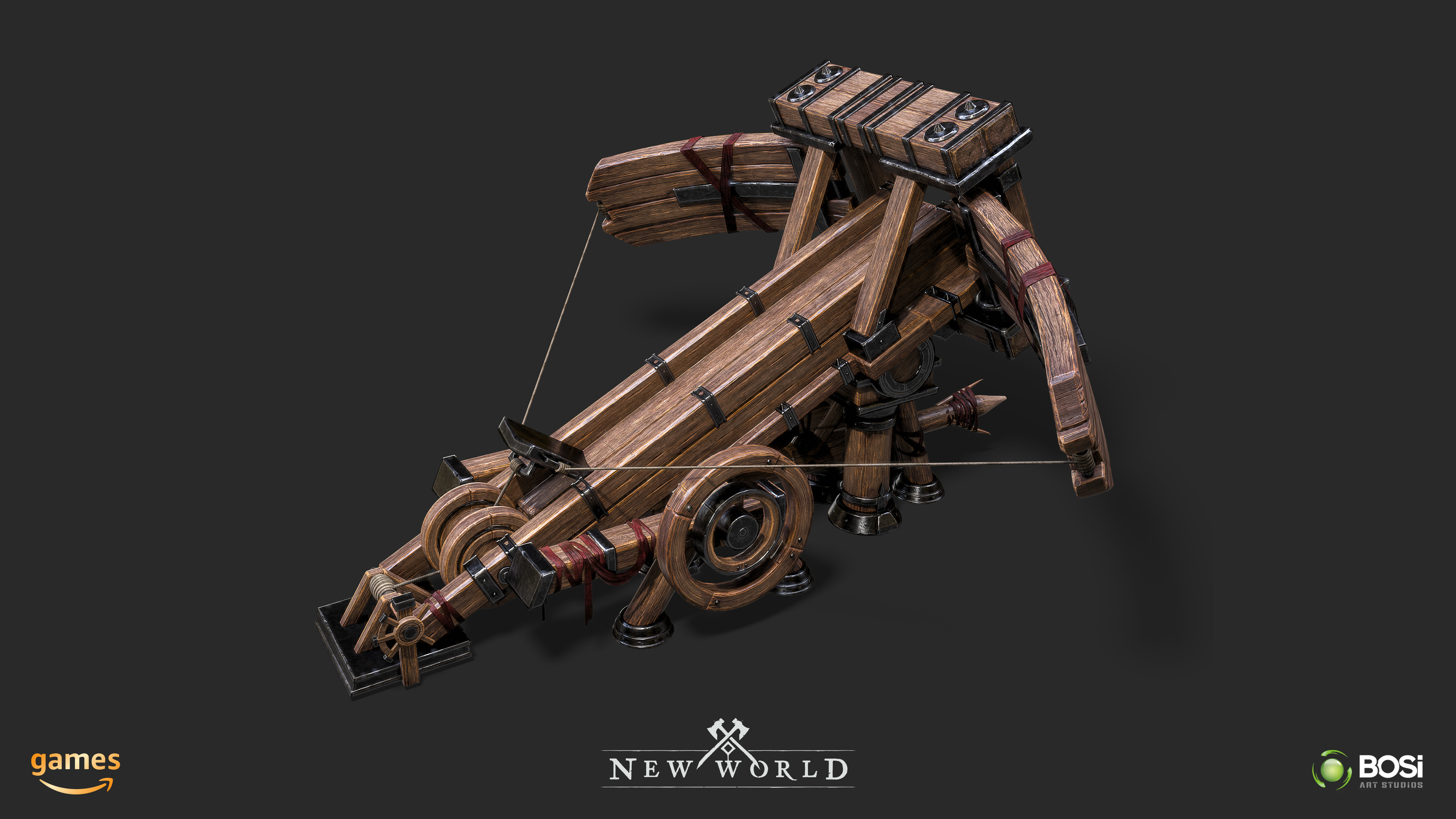The image showcases a detailed computer-generated rendering of a wooden ballista, resembling a large crossbow on wheels with mechanical features such as a cog-like handle for drawing back the bowstring. The ballista includes bent-back arms, metal strapping, and red leather wraps, but it lacks a visible projectile. The background is a mix of brownish, blackish, and gray tones, giving it a realistic old-world feel. At the bottom center of the image, the game's title 'New World' appears in white font, flanked by two overlapping white axes forming a cross. On the far left, there is the Amazon arrow logo with the word 'Games' above it, the arrow extending from the 'G' to the 'S'. On the far right, there's a 'BOSI' logo, with 'BOS' in full caps and a lowercase 'i', accompanied by a green circle featuring three small lines, though the accompanying text is illegible.